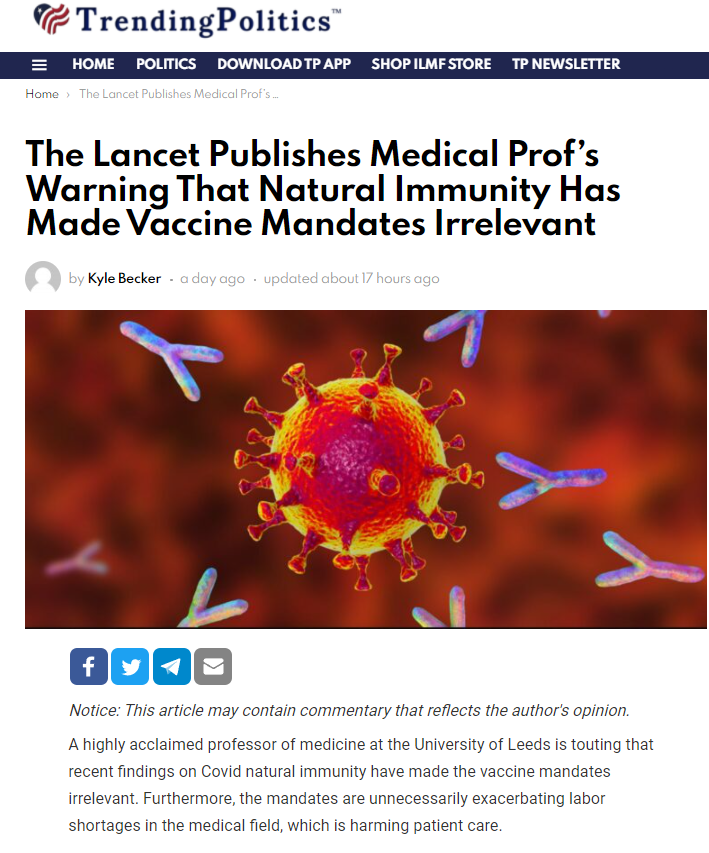The Lancet recently published findings from a group of highly esteemed medical professors, including a prominent professor from the University of Leeds, indicating that natural immunity from COVID-19 has rendered vaccine mandates unnecessary. These experts argue that the persistence of such mandates contributes to exacerbating labor shortages in the medical field, ultimately compromising patient care. This study came to light a day ago and was updated 17 hours ago.